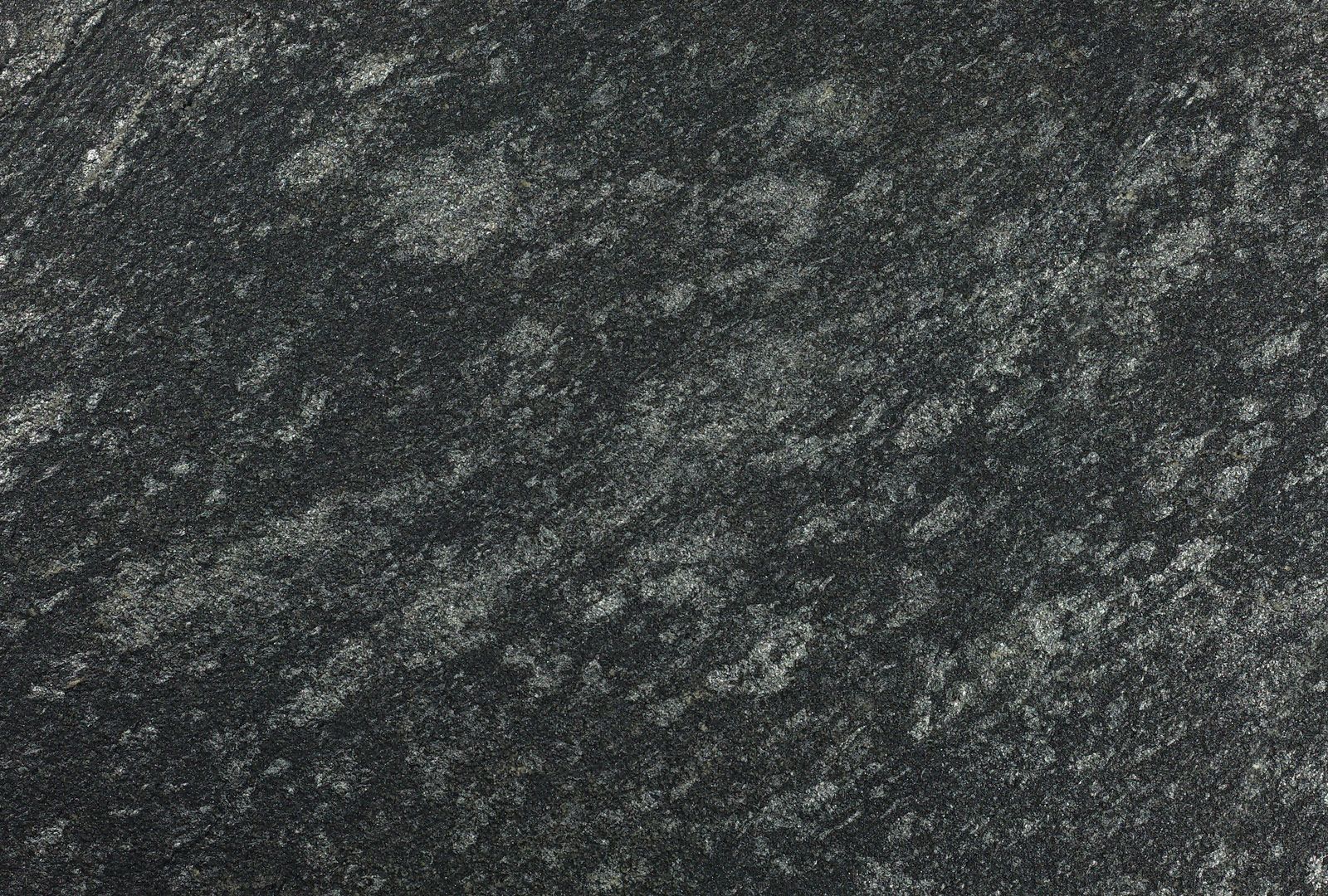The image is a black and white bird's-eye view of a large, dark grey piece of land. The surface is even, with varying textures and shades, from very dark black to pale grey and almost white in some areas. Some lighter line segments are visible in the top left corner, while scattered, irregular patches of greyish-white spots are dispersed across the rest of the surface. The absence of text or identifiable objects makes it challenging to determine whether the surface resembles a piece of rock, gravel, or ash-covered ground. Overall, the photograph captures a textured and rugged terrain, offering a detailed and abstract visual without clear context or identifiable elements.